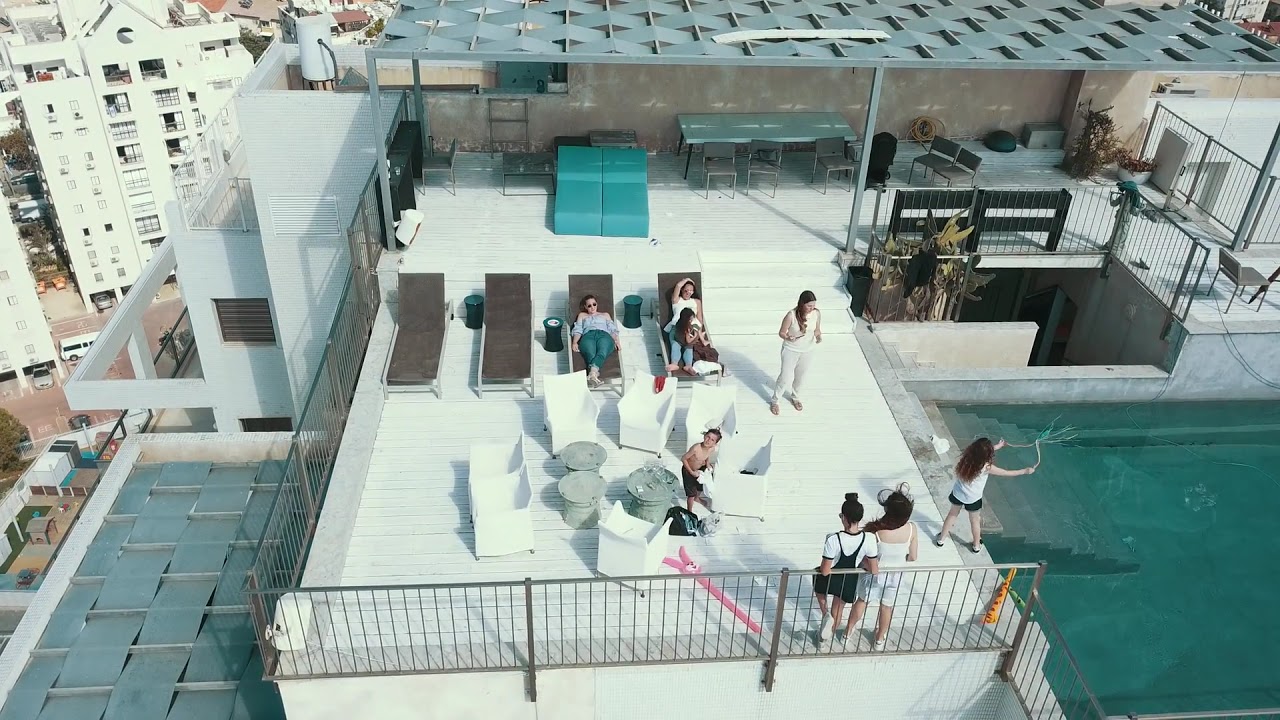The aerial photo captures a vibrant rooftop lounge area, likely atop a tall urban building, possibly a hotel. The scene is animated with approximately ten people, some standing around, while others relax on brown chaise lounges that are outfitted with dark grey mats. Off to the right side of the image, a turquoise pool glistens, with a woman nearby, with long dark hair cascading down her back, dressed in a white shirt and black shorts, seemingly creating bubbles with a bubble wand. Several blue cube-shaped seats are arranged around a table, complemented by white chairs and grey tables. A couple of women with dark hair, one styled in a bun, lean against a railing at the bottom portion of the photo, their backs turned to the camera. To the left, urban rooftops and tall apartment buildings mark the cityscape, while an intricately woven roof structure supported by thin rectangular poles provides shade to the top area of the patio. The pool area, featuring a cement staircase, further underscores the blend of relaxation and urban elegance.